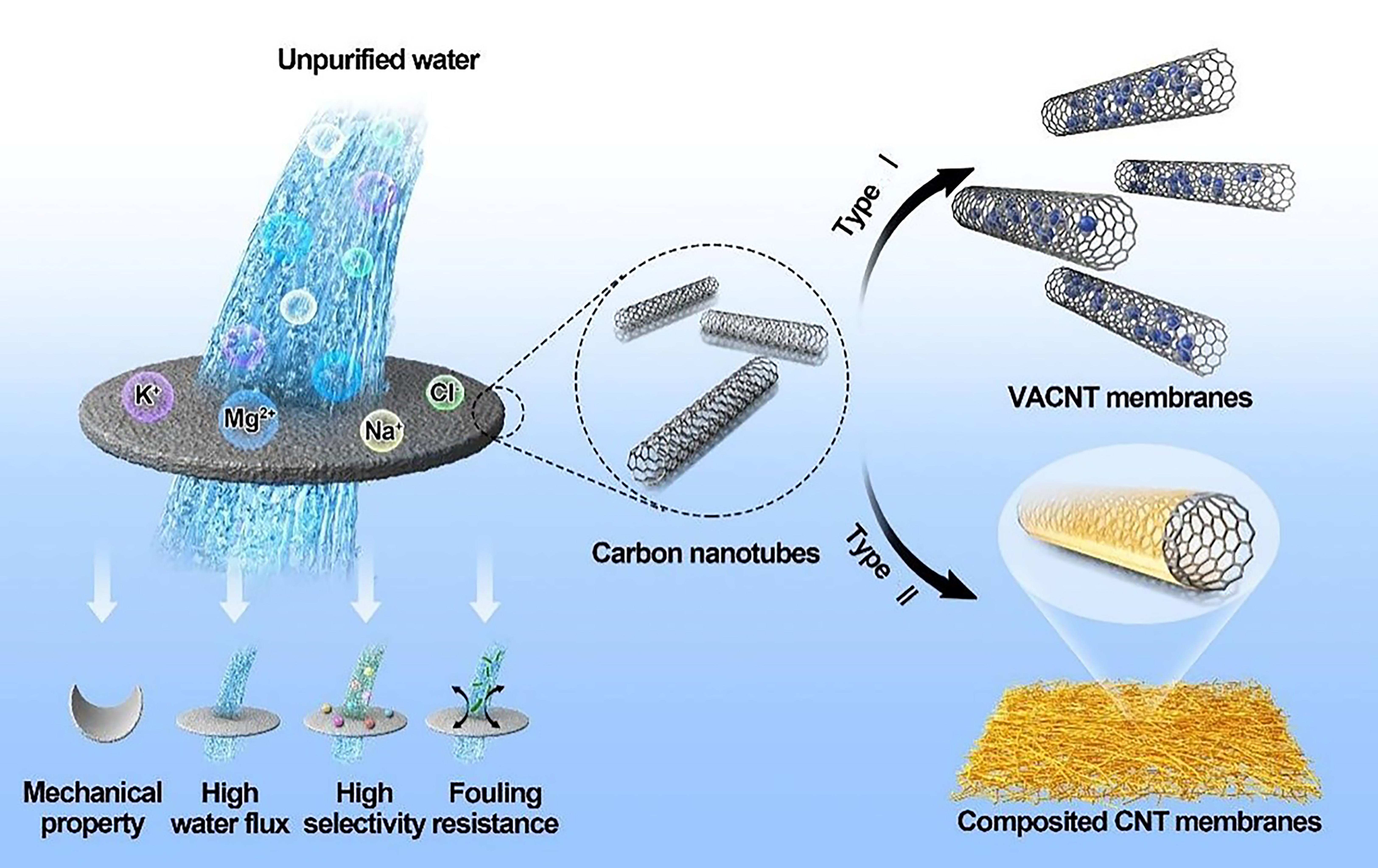The diagram features a landscape layout with a background split into two halves: the top half is white, and the bottom half is blue. On the upper left, "unpurified water" is labeled in black, with an illustration of water pouring through a gray circle that contains symbols for ions such as K+, Mg2+, Na+, and Cl-. Below this circle, four white arrows point towards silver icons labeled "mechanical property," "high water flux," "high selectivity," and "fouling resistance." In the center, the diagram highlights three carbon nanotubes, depicted as rolled-up wire structures. These nanotubes branch into two categories: the first, labeled "type one" or "VACNT membranes," and the second, labeled "type two" or "composited CNT membranes," with corresponding arrows and illustrative close-ups. The overall design of the diagram, likely from a science book, effectively conveys detailed information about the filtration and mechanical properties of carbon nanotube membranes.